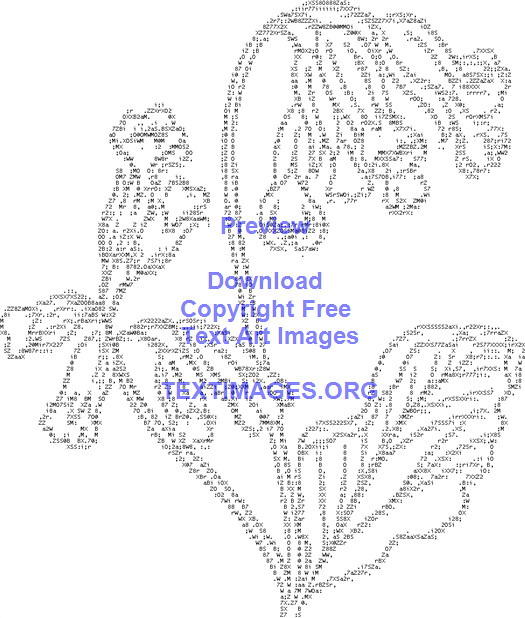The image depicts a computer-generated drawing composed entirely of small black numbers arranged to form the structure of a plant. The plant, set against a white background, features a central stem rising from the bottom center, accompanied by a leaf extending to the right. At the top, the stem curves rightward and cascades down into about six flowering buds. Additionally, another stem near the bottom extends to the left, showcasing three more flowering buds—two to the right of this stem and one to the left, with an extra bud extending sideways to the left. The entire image gives the appearance of an intricate dotted outline. The plant is centrally positioned within the image. Overlaying the drawing, in blue text, the watermark reads: "Preview Download Copyright Free Text Art Images," and "textimages.org" all in capital letters. The image has the look of an advertisement for a website specializing in text-generated art.